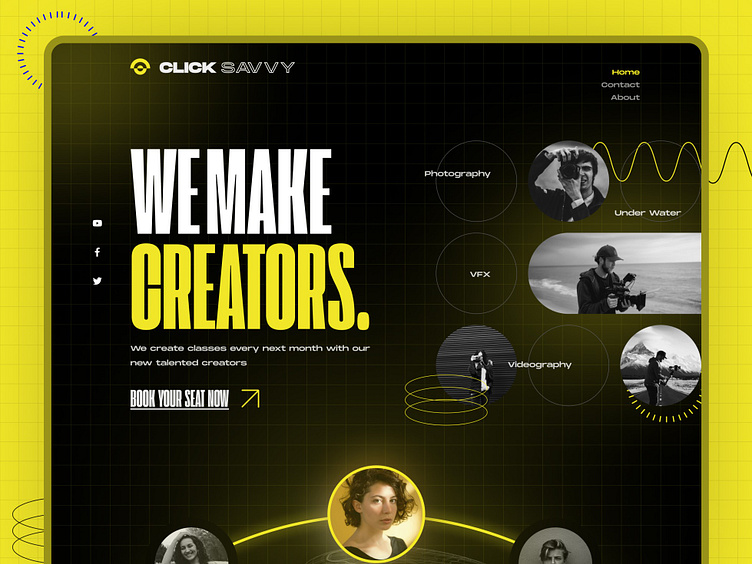The image is a mostly black and white promotional poster with elements of full color. It is basically square in shape, framed by a yellow border of squares that runs along the top, left, and right sides but leaves the bottom open. In the upper left corner, blue lines form a semicircle. The central area of the poster features a black square with grid lines, containing small blocks. At the top of this black square, text reads: "Click Savvy. We make creators. We create classes every next month with our new talented creators. Book your seat now."

In the upper right corner, navigation options labeled "Home," "Contact," and "About" are clickable. Surrounding the central text block are black-and-white images of people, likely creators, some holding cameras. The bottom center of the poster showcases a full-color image of a woman, slightly turned away but facing the camera, suggesting she might be one of the talents featured in the classes. Overall, the poster has a slick design with prominent black, white, and yellow elements, meant to attract aspiring content creators to enroll and book their seats for upcoming classes.